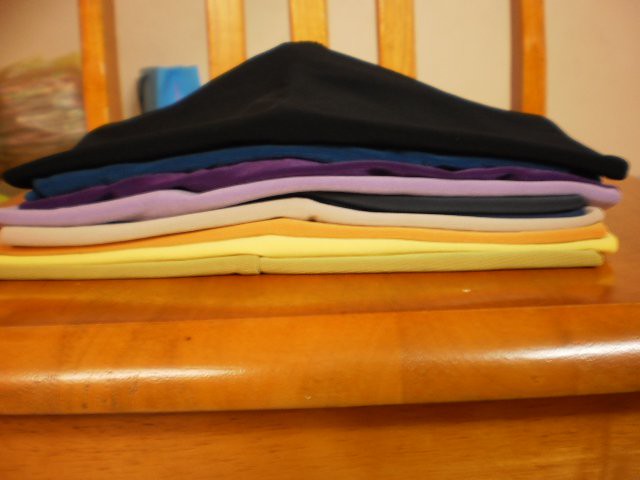This photograph depicts a neatly stacked pile of very thin, colorful fabric pieces, possibly blouses or t-shirts, folded into squares or rectangles. The fabrics are arranged on the seat of a well-defined wooden chair. The wooden chair features separate planks comprising its seat and a backrest made up of five rectangular rods. The chair’s bright brown wood contrasts with the fabrics, adding a warm, rustic element to the scene. The background is a slightly blurred beige, with a hint of something blue, possibly a bag, adding a subtle complement.

The fabrics display a rich spectrum of colors, starting from the bottom: a dark yellow piece at the base, followed by a bright yellow, a light orange, a beige, a dark blue-gray, a light purple, a dark purple, a blue, and topped with a black piece that appears slightly pointed, giving the stack a bit of a triangular shape at the top. The orderly arrangement and vivid colors make the image visually striking, capturing the textures, hues, and the organized serenity of folded garments.